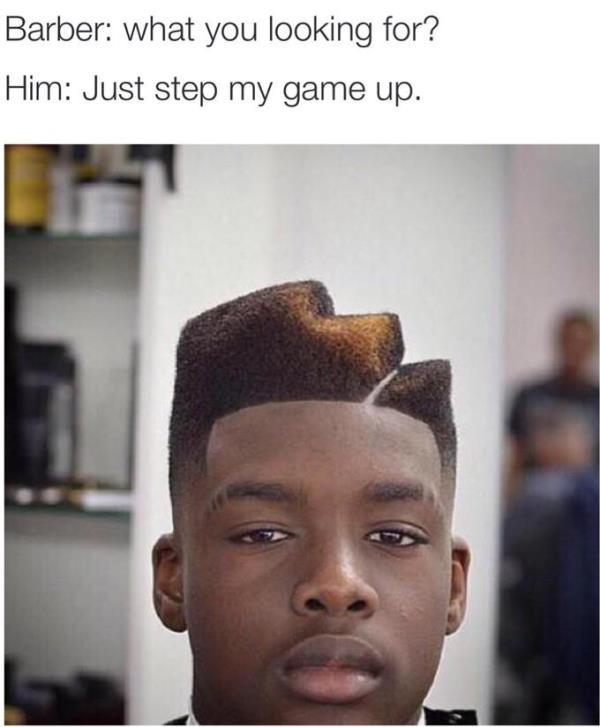This image, reminiscent of a meme, features two lines of dark, almost black, text at the top: the first reading, "Barber: What are you looking for?" followed by, "Him: Just step my game up." Below the text is a detailed photograph of a black man at a barbershop. His freshly cut hair is styled into a distinct fade with stair-step-like cuts at the top, and a stylish line etched into the left side of his head. The man's face, dark-skinned with a highlighted streak of lighter brown through the middle of his hair, looks directly at the camera. The background is blurred but indicates a typical barbershop setting, with indistinct hair products visible and a person wearing a black shirt slightly off to the right.